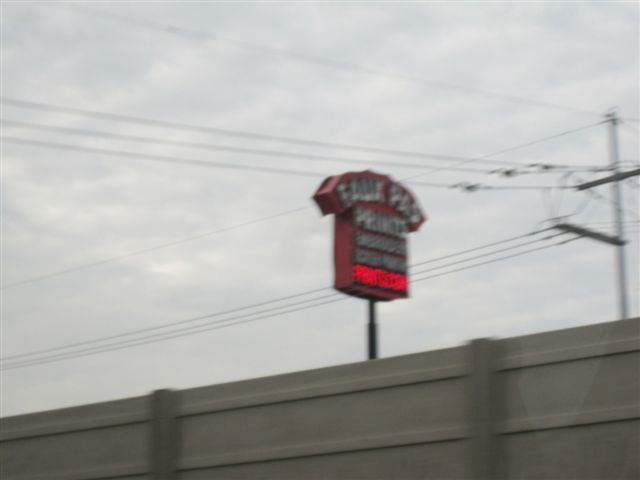This blurry color snapshot, taken outdoors on a cloudy day with a sky filled with white and dark gray clouds, captures a scene dominated by a tilted, gray sound wall stretching from the lower left-hand corner to the center right side of the image. Behind the sound wall stands a tall, rectangular sign with a curved banner on top, resembling a paw print. Though the sign is mostly illegible, the upper part features a white background with a black border and a bright red illuminated section at the bottom. Also visible are an electrical pole with numerous wires extending across the image. The cement structure beneath the sign suggests it could be associated with either a pet-related business or a printing shop. The overall composition is blurred, adding to the mystery and ambiguity of the scene.